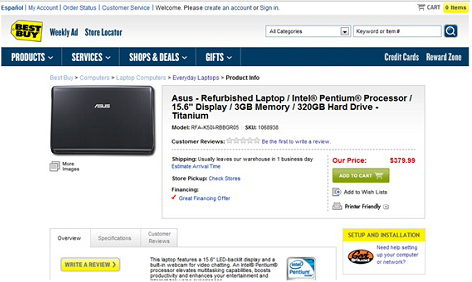This screenshot showcases an old Best Buy website layout from approximately 10 years ago. On the top left side of the header, the familiar Best Buy logo is prominently displayed on a yellow price tag. Adjacent to the logo, navigational links for the "Weekly Ad" and "Store Locator" are visible. The same row also hosts an "All Categories" drop-down menu and a search bar equipped with a blue button featuring a magnifying glass icon. 

Beneath this header, a navy blue stripe includes four main tabs: "Products," "Services," "Shop," "Deals & Gifts." The main content of the page features a detailed listing for an Asus refurbished laptop. The laptop, positioned on the left side of the page, boasts an Intel Pentium processor, 15.6-inch display, 3GB of memory, and a 320GB hard drive. The device is finished in titanium gray.

To the right of the laptop image, the model number (SKU 1066506) is specified, along with its price of $379.99, which is highlighted in red. Directly beneath the price is a green "Add to Cart" button, encouraging immediate purchase.

Towards the bottom right of the page, a smaller box titled "Setup & Installation" features the Geek Squad logo—an oval shape with its upper half in orange and the lower half in black, emblazoned with the words "Geek Squad." Directly below this box, another section provides options for "Overview," "Specifications," and "Customer Reviews," complete with a yellow "Write a Review" button for user-generated content.